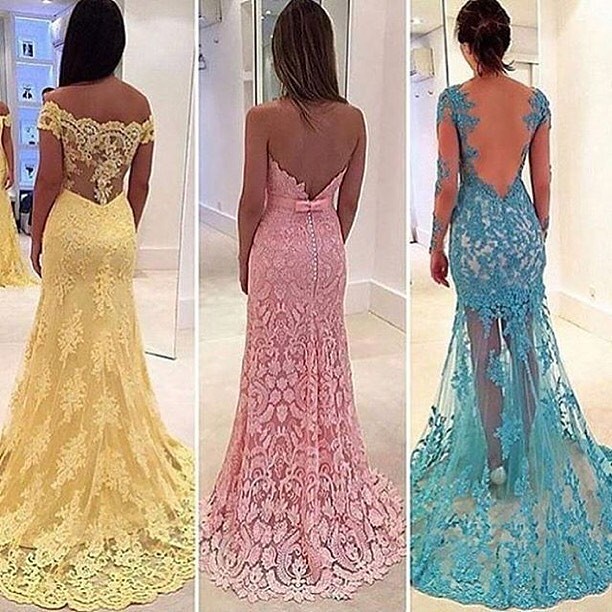In this meticulously detailed photograph collage set in a white-background dressing room, three elegant women showcase enchanting gowns exuding a timeless charm. The leftmost woman, possessing dark skin and long dark hair, is adorned in a stunning yellow gown. This gown features off-the-shoulder short sleeves composed entirely of intricate yellow lace, which elegantly cascades down her back, flowing into a voluminous yellow skirt overlaid with matching lace. She stands gracefully before a mirror, reflecting her resplendent attire.

The middle woman, with tan skin and brown hair accentuated with subtle yellow streaks, dazzles in a soft blush pink, strapless gown. This gown descends into a V shape on her back, adorned with a delicate pink bow at the small of her back, and detailed with a row of small white buttons. The lace overlay extends to the edges of the gown, providing a charming contrast.

The rightmost woman, exhibiting lighter skin and dark hair styled in an elegant updo, wears a striking blue gown. The dress is characterized by its long sleeves made almost entirely of delicate lace, which sparsely decorates her arms with blue floral patterns. The gown provides a peekaboo effect with an exposed back and features a solid blue underdress that transitions into a sheer lace from the upper thighs, adorned with intricate blue decorations extending to the floor. Together, these women exemplify a harmonious blend of grace and sophistication, each gown uniquely complementing their individual beauty.